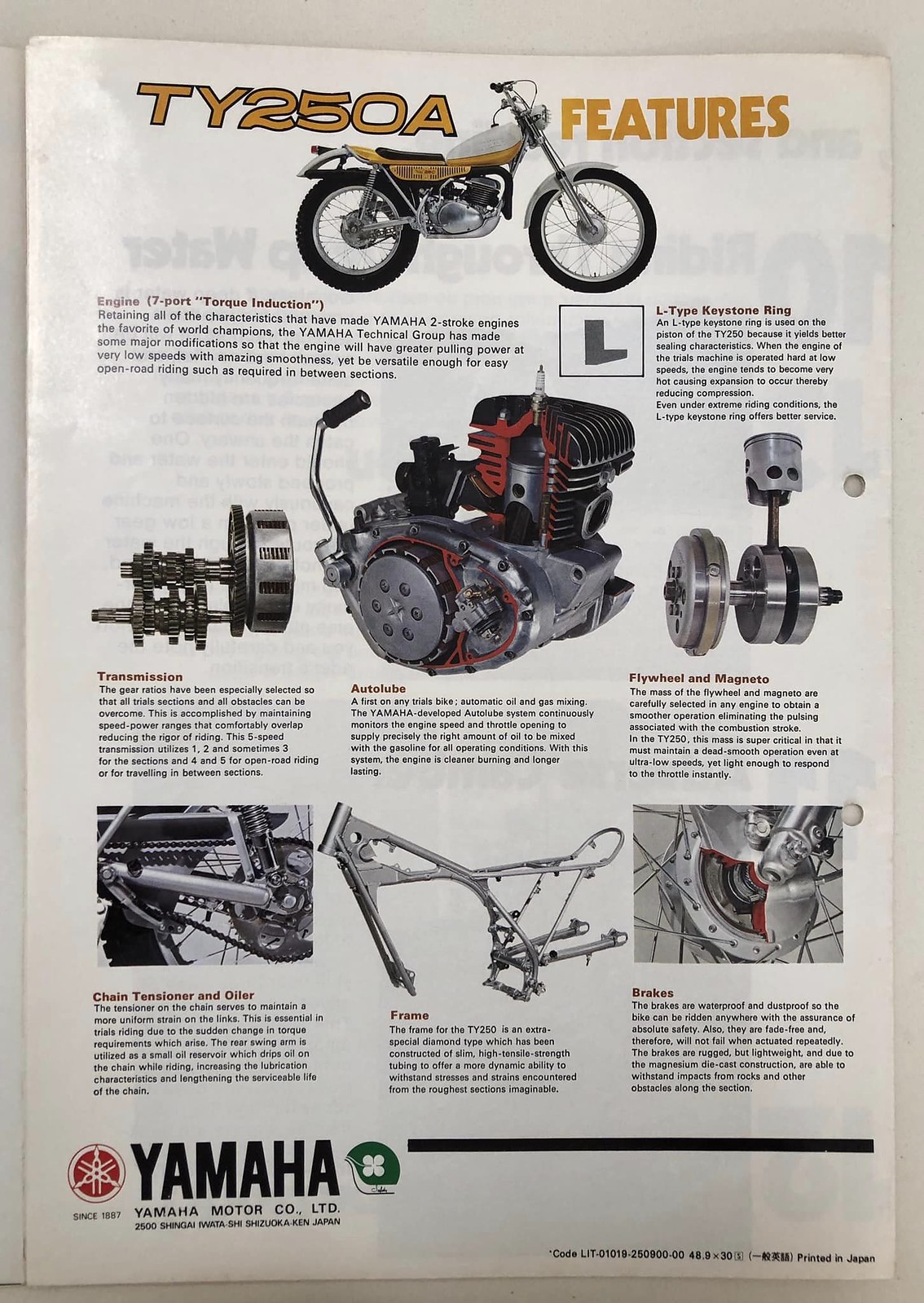This advertisement, seemingly taken from a magazine, showcases a vintage Yamaha TY250A motorcycle, likely from the 1970s or 1980s. The motorcycle, adorned in yellow and white with black accents and white fenders, is prominently displayed at the top, with its model name "TY250A Features" highlighted in a yellow font. The centerpiece of the ad is a detailed die-cast, exploded view of the motorcycle engine, revealing intricate internal mechanics. Key components like the crankshaft, piston, and gear set are spotlighted on the right and left, respectively. The swingarm, drivetrain, frame, and brakes are also depicted in various corners of the illustration. Despite the thorough detailing, the descriptive text accompanying each part is not legible due to the photo being taken from too far away. At the advertisement’s bottom left, the Yamaha Motor Co. LTD logo is visible next to the red Yamaha tuning fork symbol, alongside a green and white half helmet, affirming its authenticity and origin from Japan.